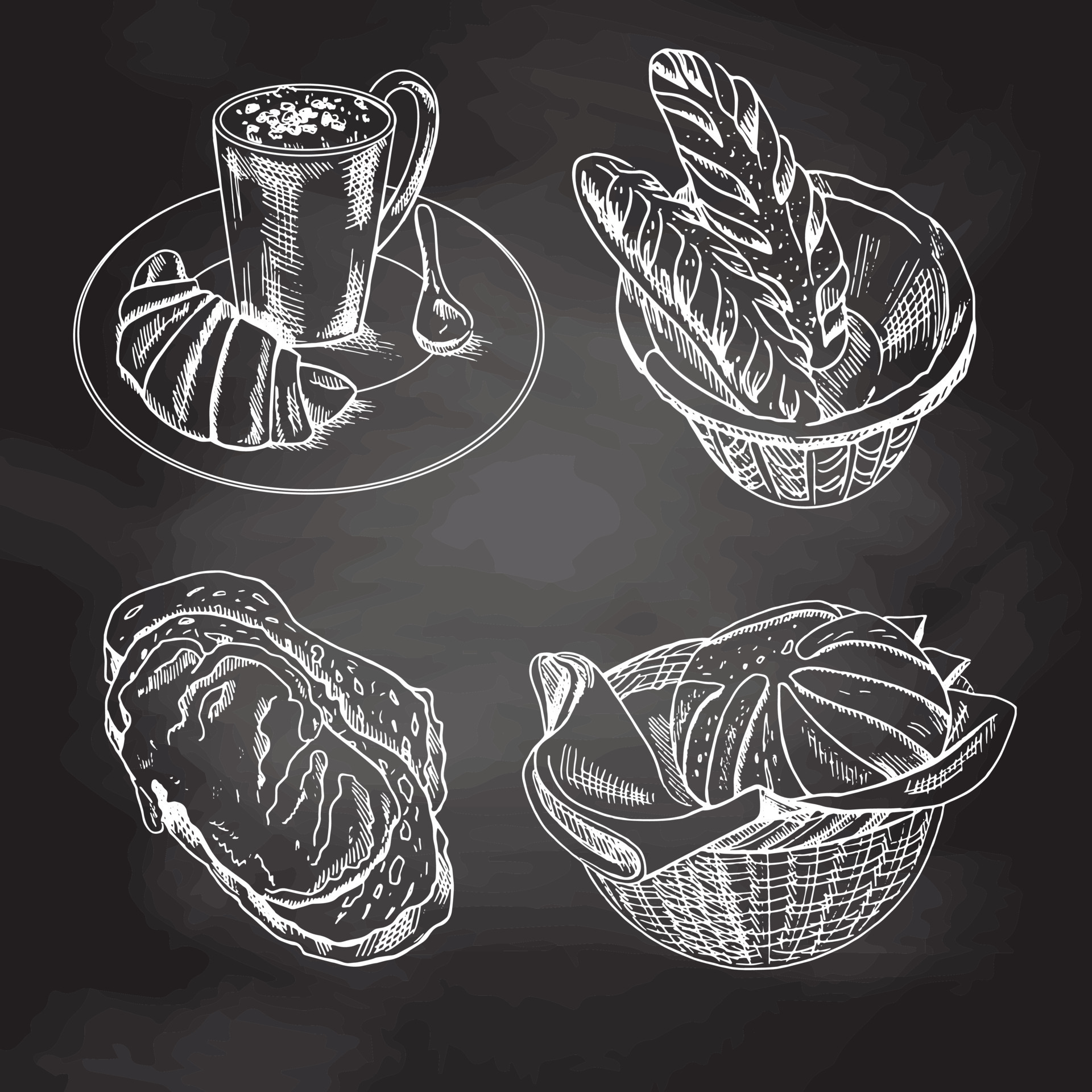The image displays a black and gray chalkboard-like surface, transitioning from a darker edge to a lighter gray center with a swirly pattern typical of chalk erasures. Four white chalk sketches of food items, arranged symmetrically, occupy the square frame. The upper left features a mug with a handle, set on a saucer, accompanied by a croissant and a spoon. The upper right depicts two long, braided loaves of bread resting in a basket. The lower right contains a round loaf of bread placed on a napkin inside a round basket. The lower left shows two steaks stacked diagonally. Each drawing is created with white lines, combining to form a cohesive and visually appealing chalkboard art piece.